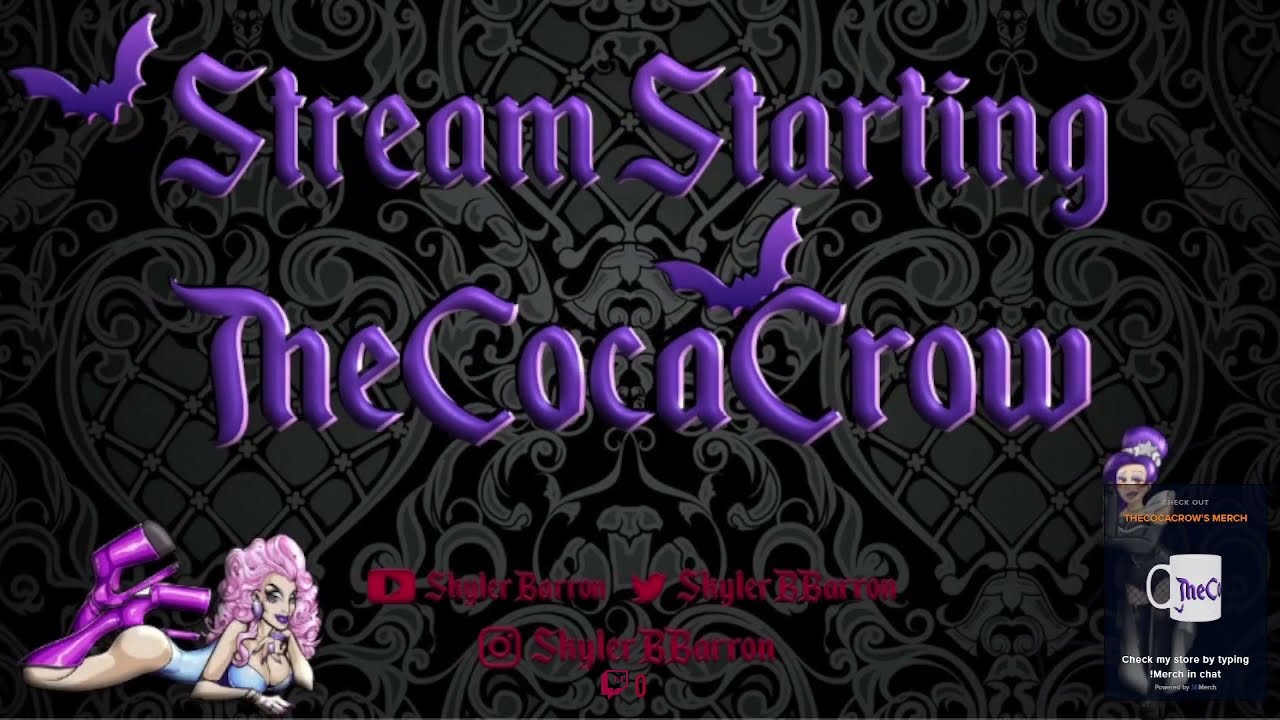This illustration features a promotional design with a gothic aesthetic and several eye-catching elements. Dominating the top of the image is a bold, almost 3D blue font that reads "Stream Starting." Below this, the text "The Cocoa Crow" is highlighted, embellished with a purple bat on the top left, and another bat hovering over the second 'C' in 'Crow'. The background maintains a gothic theme with symmetrical grey patterns against a black backdrop, adding depth and mystery to the design.

On the bottom left, an animated woman lies on her stomach, clad in revealing attire that includes a bathing suit or lingerie. Her pose accentuates her bent knees, bringing her high-heeled stilettos close to her buttocks. Details such as her exposed breasts and minimal clothing contribute to her seductive appearance. Her striking pink hair and purple, knee-high boots with exaggerated heels make her a focal point of the illustration.

To the right of the image is another woman with blue hair, accompanied by some white text and symbols, though the specifics are hard to discern. The symbols likely include social media icons like YouTube, Twitter, and Instagram, suggesting a digital or streaming context for the promotion. Additionally, a white coffee cup with undecipherable text adds to the array of elements on the right side. The entire design is layered over a backdrop rich with gothic style grey and black prints, incorporating hearts and other intricate patterns to complete the immersive visual theme.